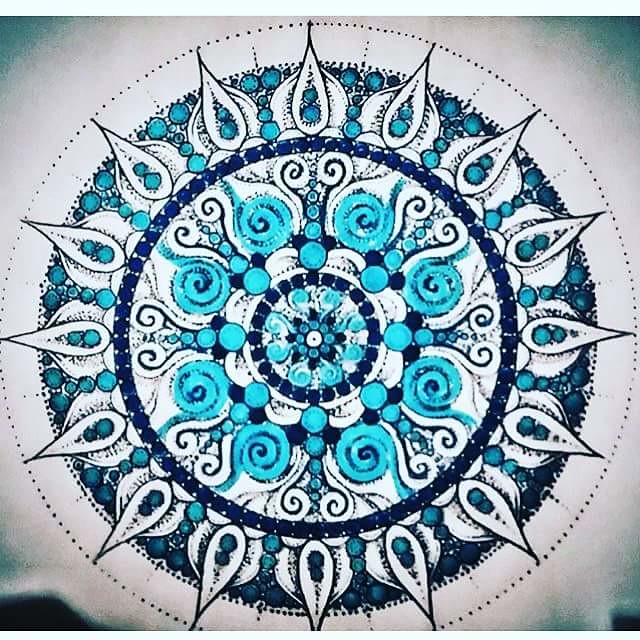This image features an intricate mosaic artwork set against a pristine white background. Dominating the composition is a large, circular pattern meticulously crafted from black dots. Within this prominent circle lies a mesmerizing design characterized by concentric circles that transition from blue to white, creating a striking visual effect. The innermost circle is a pure white, bordered by a dense ring of blue dots. Radiating from the core, the design showcases a series of teardrop-shaped motifs in varying shades of blue, interspersed with dark blue elements that enhance the depth and complexity of the artwork. Swirling patterns and delicate curlicues add to the enchanting, almost hypnotic, quality of this mosaic, culminating in a harmoniously balanced and visually captivating piece.